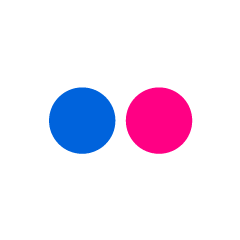The image features a minimalistic composition set against a stark white background. Positioned centrally are two perfectly round circles; the one on the left is a rich royal blue, while the one on the right is a vibrant pinkish-red. Both circles are identical in size, roughly comparable to a dime. The image is devoid of any text, additional markings, or shadows, emphasizing the pure, unembellished nature of the circles. The simplicity and clarity of the design make the two circles—one blue and one pinkish-red—the sole focal points of the image.